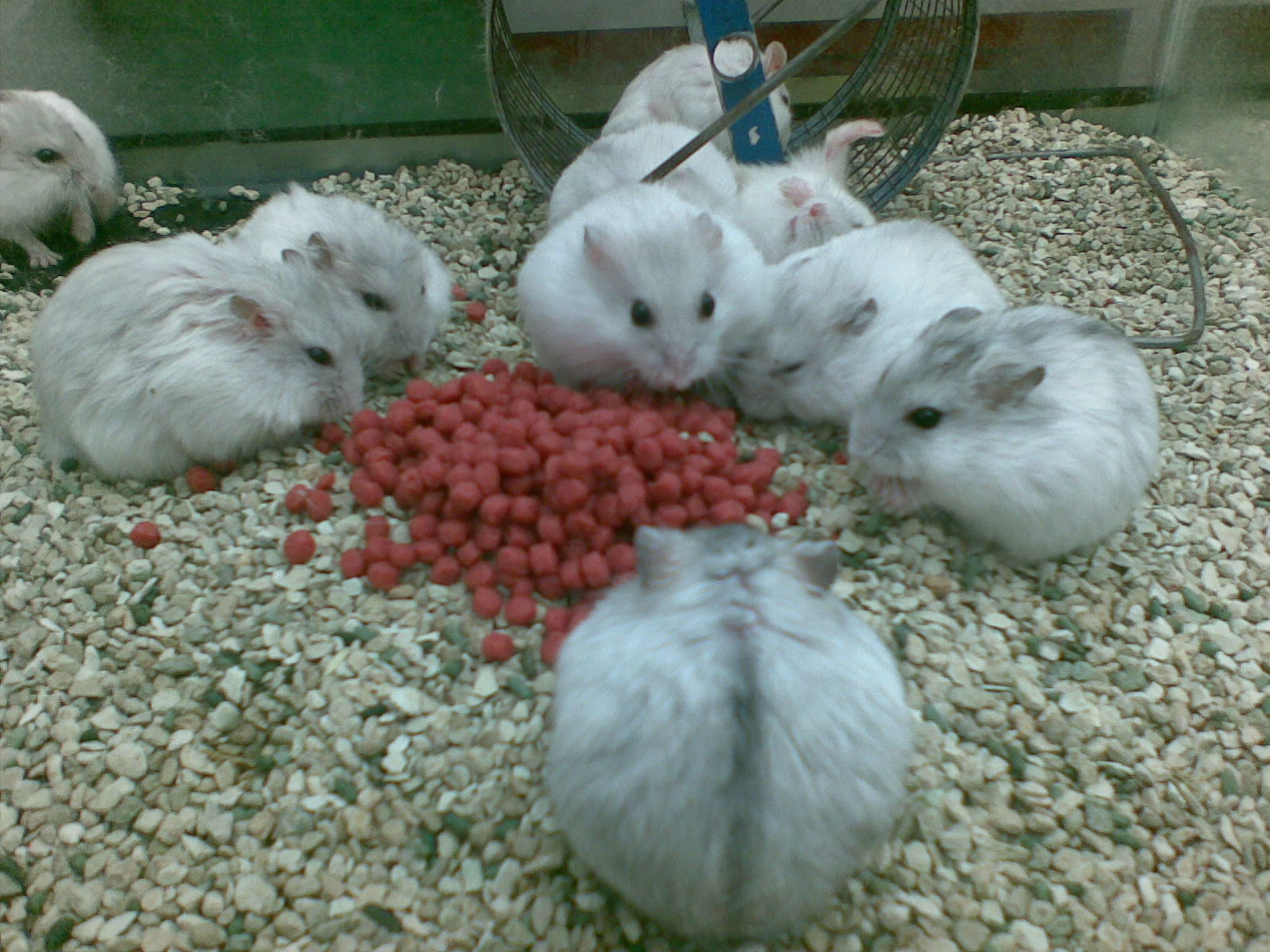This photograph showcases a captivating and warm scene of 10 white hamsters, some adorned with a faint light gray stripe running along their spines, within a glass-walled aquarium. The floor of their enclosure is covered with small, soft, pebble-like gravel. Centrally positioned in a semicircle, six of the hamsters are contentedly munching on a pile of reddish food pellets, creating an inviting and wholesome atmosphere. In the background, one hamster is energetically exercising on a wheel, while another appears to be scratching itself in the top left corner. There's also a hamster lying on its back, seemingly enjoying the soft pebbles, with another one standing nearby, curiously observing its surroundings. This adorable and heartwarming scene evokes a sense of warmth and fuzziness.